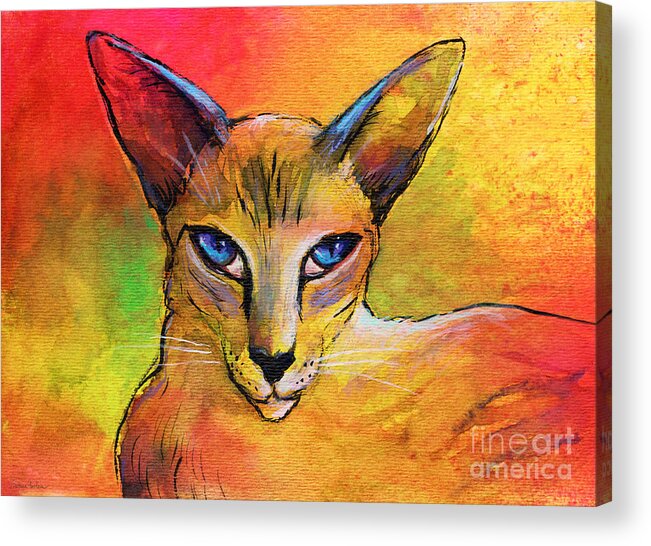The image is a detailed artwork on an unframed wrapped canvas, featuring a cat painted in shades of orange, yellow, and a touch of green with a blended background that mirrors these colors. The cat, depicted from the shoulders up and facing forward, has striking bright blue, angular eyes, and long, pointed ears. Its nose and muzzle, outlined in black with whiskers emerging from black dots, add to the detail, and its body extends towards the right edge of the canvas. Notably, the cat's muzzle is more white compared to the rest of its body. The bottom right corner of the artwork bears a translucent white watermark that reads "Fine Art America." The sides of the canvas are also painted, ensuring the artwork's colors wrap fully around.